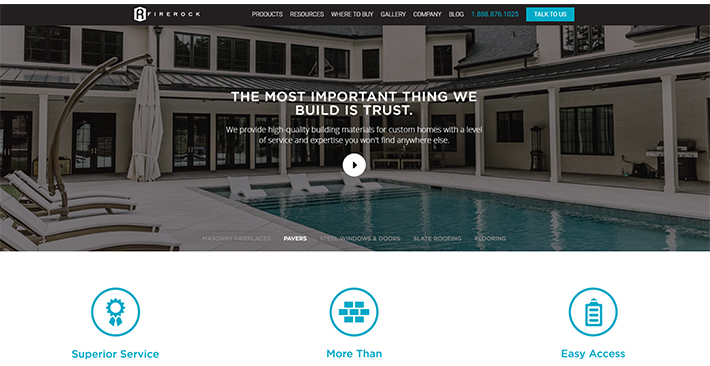The FireRock website showcases their dedication to providing high-quality building materials for custom homes, accompanied by unparalleled service and expertise, encapsulated by their slogan, "The most important thing we build is trust." The website features a sleek design with convenient navigation options including sections for products, resources, where to buy, gallery, company, and blog. A prominent phone number in blue is available for immediate customer support under the "Talk to Us" link.

The centerpiece image on the webpage is an expansive, in-ground pool, evocative of a luxurious villa or high-end hotel. The pool area is adorned with built-in lounge chairs positioned strategically at the steps for a relaxing in-water experience. Additional lounge chairs line the sides of the pool, each paired with large umbrellas that can be adjusted to provide shade, ensuring comfort for those wanting to avoid direct sunlight. The grandeur of the setting suggests it's designed for hosting numerous guests, highlighting the lavish space and premium materials that FireRock prides itself on delivering.